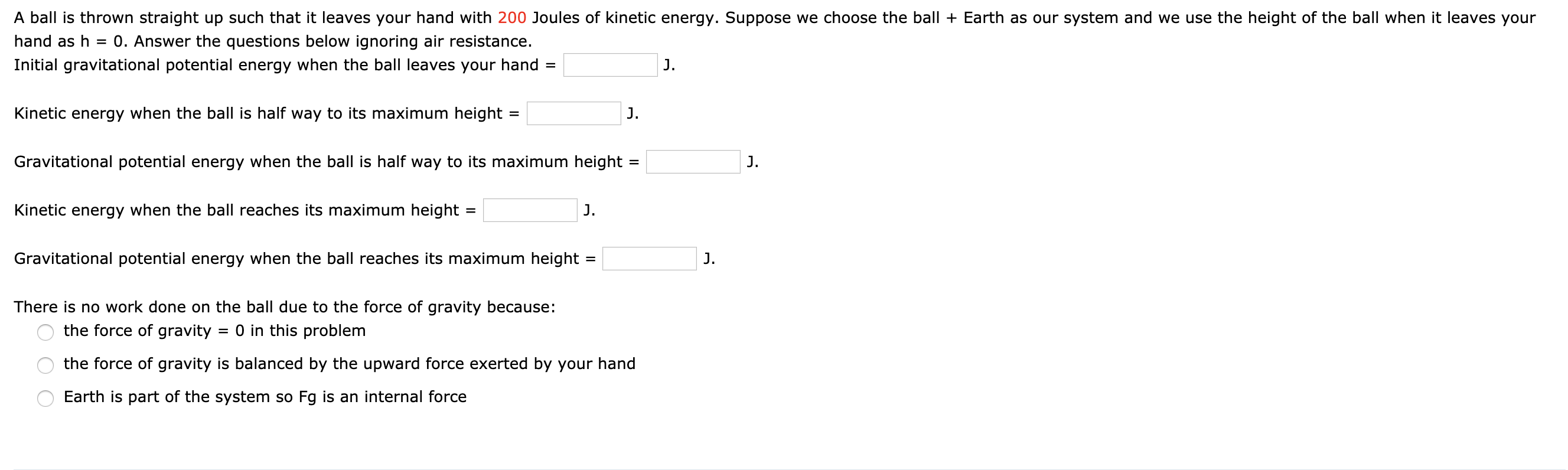The image appears to be a screenshot from a science or math quiz, focusing on a physics problem involving kinetic energy and gravitational potential energy. The background is white, with text in black, and the only splash of color is "200 joules" written in red. The problem reads: 

"A ball is thrown straight up, leaving your hand with an initial kinetic energy of 200 joules. Suppose we choose the ball and the Earth as our system, and set the initial height, h = 0, at the point where the ball leaves your hand. Consider the following questions, ignoring air resistance:

- Initial gravitational potential energy (when the ball leaves your hand) = __ J
- Kinetic energy (when the ball is halfway to its maximum height) = __ J
- Gravitational potential energy (when the ball is halfway to its maximum height) = __ J
- Kinetic energy (when the ball reaches its maximum height) = __ J
- Gravitational potential energy (when the ball reaches its maximum height) = __ J

Additionally, a multiple-choice question follows: 'There is no work on the ball due to the force of gravity because:'
- The force of gravity equals zero in this problem.
- The force of gravity is balanced by the upward force.
- Earth is part of the system, so Fg is an internal force."

This detailed scenario clearly sets up a physics problem addressing the conservation of energy during the vertical motion of a ball.